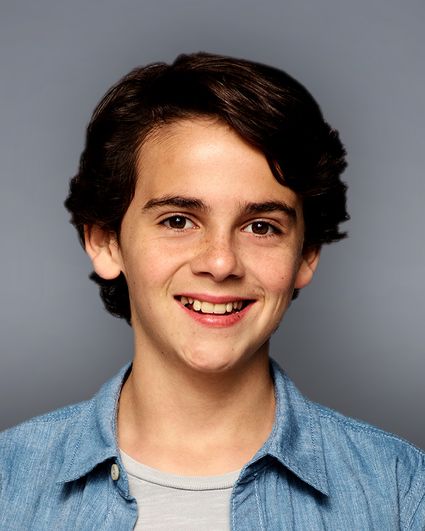The image portrays a teenage boy, approximately 15 years old, with dark, wavy black hair that cascades down to his ears and dark eyebrows. He has a cheerful expression, smiling openly with his upper teeth visible, accentuating freckles on his nose and upper cheeks. He is dressed in an unbuttoned light blue denim shirt with a button on the collar, layered over a lighter t-shirt that appears to be a mix of blue and gray shades. The backdrop is a simple, light gray, consistent with professional portrait backgrounds, evoking the style of a high school yearbook photo. The portrait is in color and professionally taken, capturing the boy's friendly demeanor.